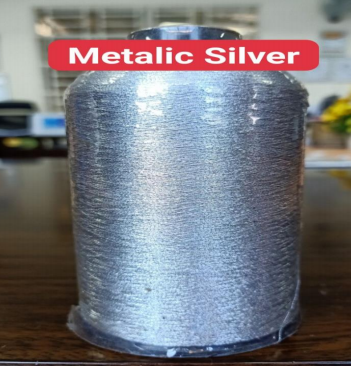In the image entitled "Metallic Silver," prominently displayed in white letters on a red banner just below the top of the image, a spool of metallic silver twine is the main focus. The twine, which is wrapped in plastic, sits on a black base and is cylindrical in shape, approximately four to five inches tall. A black circular opening at the top of the spool can be seen above the label, which reads "Metallic Silver." The spool is centrally positioned on a wooden table. Behind the table, the background reveals a setting that appears to be indoors, possibly an office or industrial environment, featuring large windows and various appliances. The image features a color palette including shades of black, brown, silver, gray, red, blue, yellow, and green.